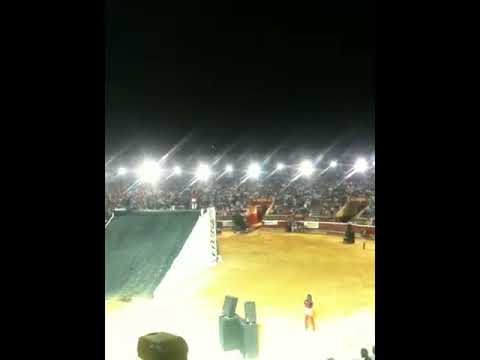This image depicts a nighttime event within an expansive stadium, likely a monster truck rally or motocross show. Dominating the left center of the frame is a towering, white-framed ramp accented in green, aiming skyward, suggesting an imminent high-flying jump. Below the ramp, the ground is a rich brown dirt, typical of such arenas. To the right of the ramp, the dirt arena stretches out, bounded by a blurry mass of spectators cloaked in shadowed obscurity, their forms indistinct against the distant stands. These stands are intermittently illuminated by intense white spotlights, piercing the darkness of the night sky that blankets the top third of the image.

A striking red banner encircles the arena, creating a vivid contrast with the brown dirt and darkened audience. Among the few discernible figures, a woman dressed in white shorts and a purple t-shirt stands out near the ramp's base, beside some speakers. The position of the camera, seemingly from within the bleachers, frames this bustling scene of anticipation and energy, highlighting the crowd gathered to witness the spectacle of airborne feats to come.